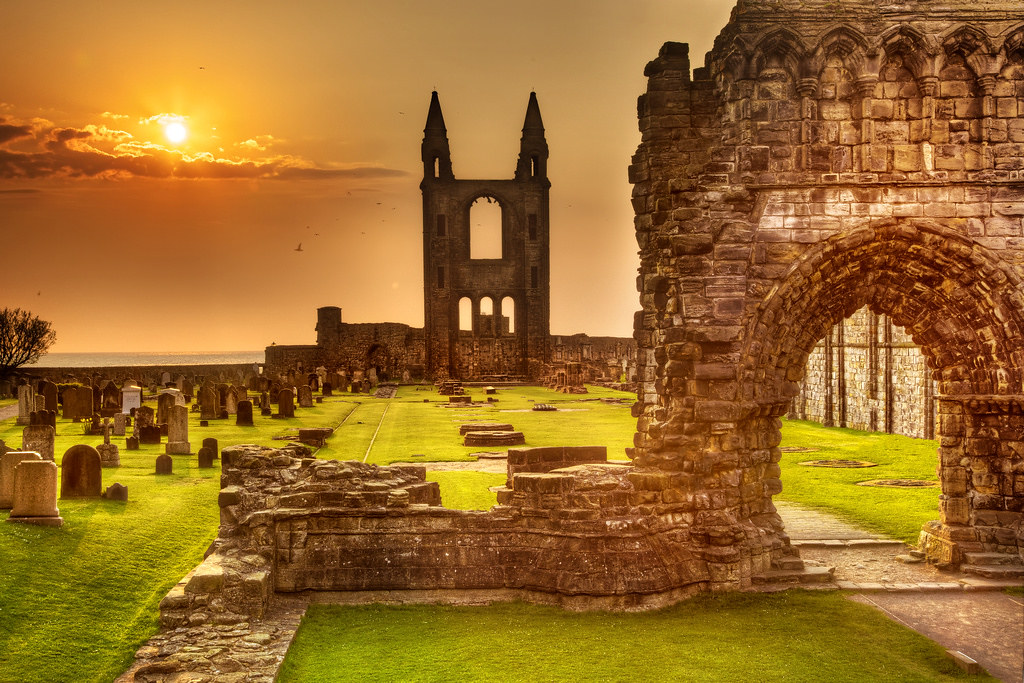This photograph captures the evocative ruins of an ancient structure, likely a historic heritage site, enveloped in the golden hues of a setting sun. On the right side of the image, a prominent arched gateway, constructed from aged brown bricks and rocks, stands resilient, its surface partially covered in moss. Beyond this entrance, the ground is carpeted with carefully manicured green grass, leading the eye to additional building ruins in the distance, including what appear to be two towers reminiscent of a gothic church. On the left side of the image, a number of tombstones—varying in color, size, and disorganized placement—suggest a graveyard, adding to the scene's aged mystique. The sky above is a dramatic canvas of orange-tinted clouds, with the sun hovering low on the left, casting a warm, orange-yellow glow over the entire landscape.